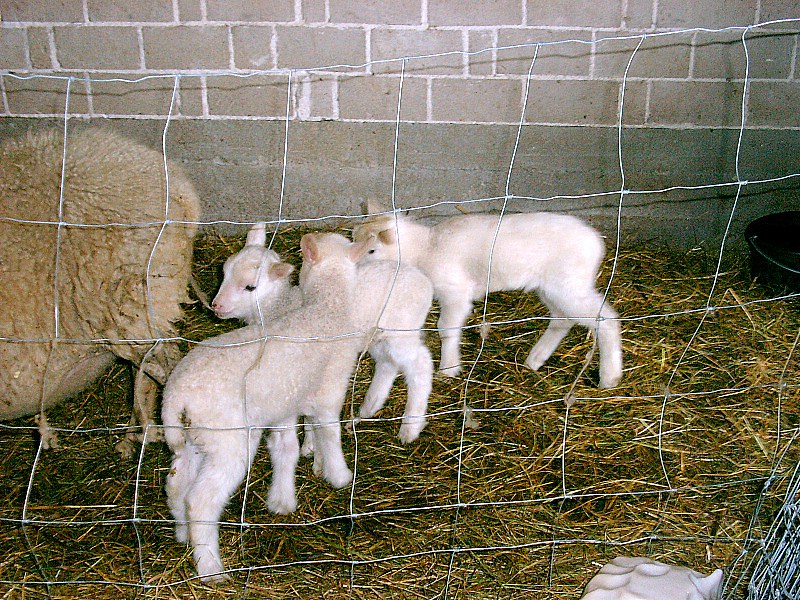The photograph showcases a pen containing three baby sheep, or lambs, with light tan to almost white coats, contrasted against the partially visible, more tan-brown outline of what seems to be their mother. The pen is bordered by a wire fence, with chain-link fencing visible in the bottom right-hand corner and a wall of concrete blocks at the back. The pen floor is strewn with hay. Within the image, two of the lambs are positioned towards the back, both facing left. The third lamb, closer to the front, faces slightly away from the camera with its head resting on the back of one of the other lambs. A bowl, possibly for water, sits in the middle right of the photo.